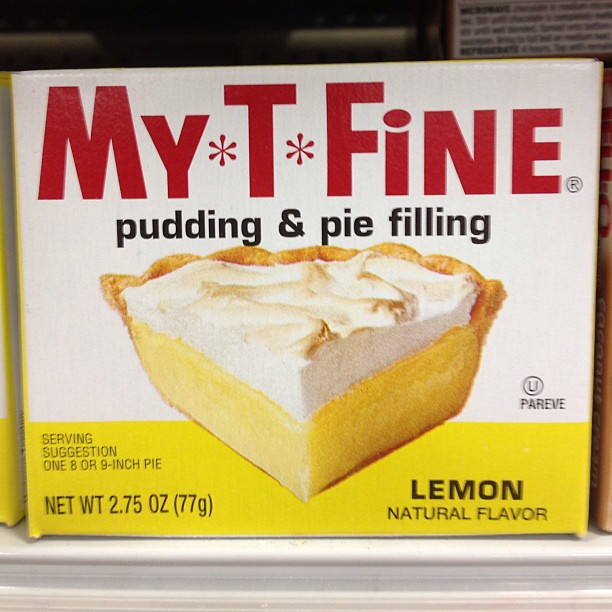This photograph showcases a vintage-looking box of My-T-Fine pudding and pie filling. The box features a white background with a yellow strip at the bottom. Prominently displayed at the top is the brand name "My-T-Fine," spelled M-Y, followed by a star, then the letter T, another star, and finally the word "Fine" in large, bold red letters. Below the brand name, "Pudding and Pie Filling" is printed in black text. The packaging includes an image of a lemon meringue pie slice, with a browned, torched meringue topping and a lemon filling underneath. A pie crust surrounds the slice. To the right of the pie image, a circle with a 'U' inside indicates the kosher certification, alongside the word "PAREV" and suggestions for serving an 8 or 9-inch pie. The product weight is specified as 2.75 ounces (77 grams). The bottom right corner of the packaging also notes "lemon natural flavor" in black text.